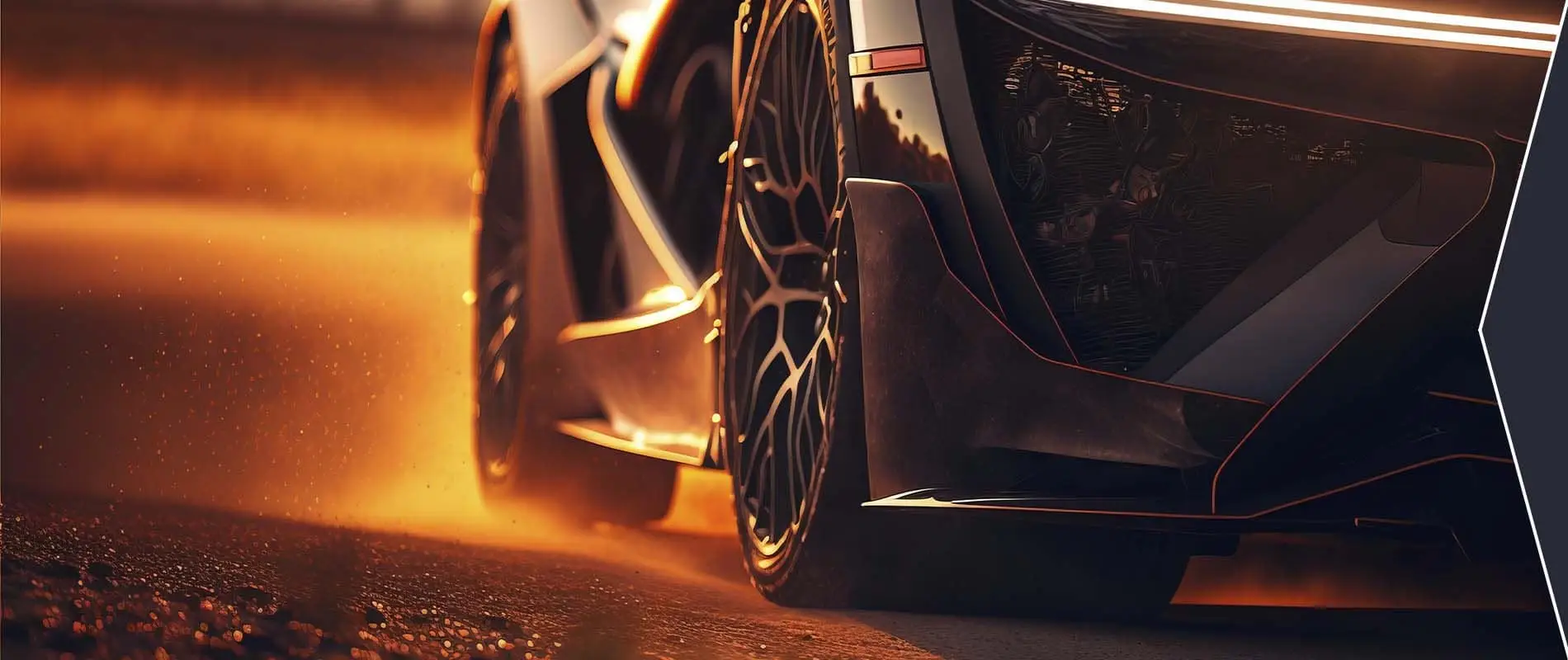This image captures the sleek, lower half of a futuristic, concept car reminiscent of the Batmobile. Photographed from a low angle close to the ground, the picture focuses on the right side of the vehicle, highlighting its intricate design details. The car sports broad, strikingly branched wheels with intricate, spiraled rims, and its exterior is a gleaming, dark gray-black with subtle reflections of an orangey sunset. The wet, glistening road beneath the car, along with the dust and rocks being kicked up by the tires, suggests motion. Surrounding shrubbery reflects on the shiny bumper, indicating a forest setting. The scene is dramatically lit by golden sunlight, adding to the impression of a high-speed journey through a serene, natural landscape.